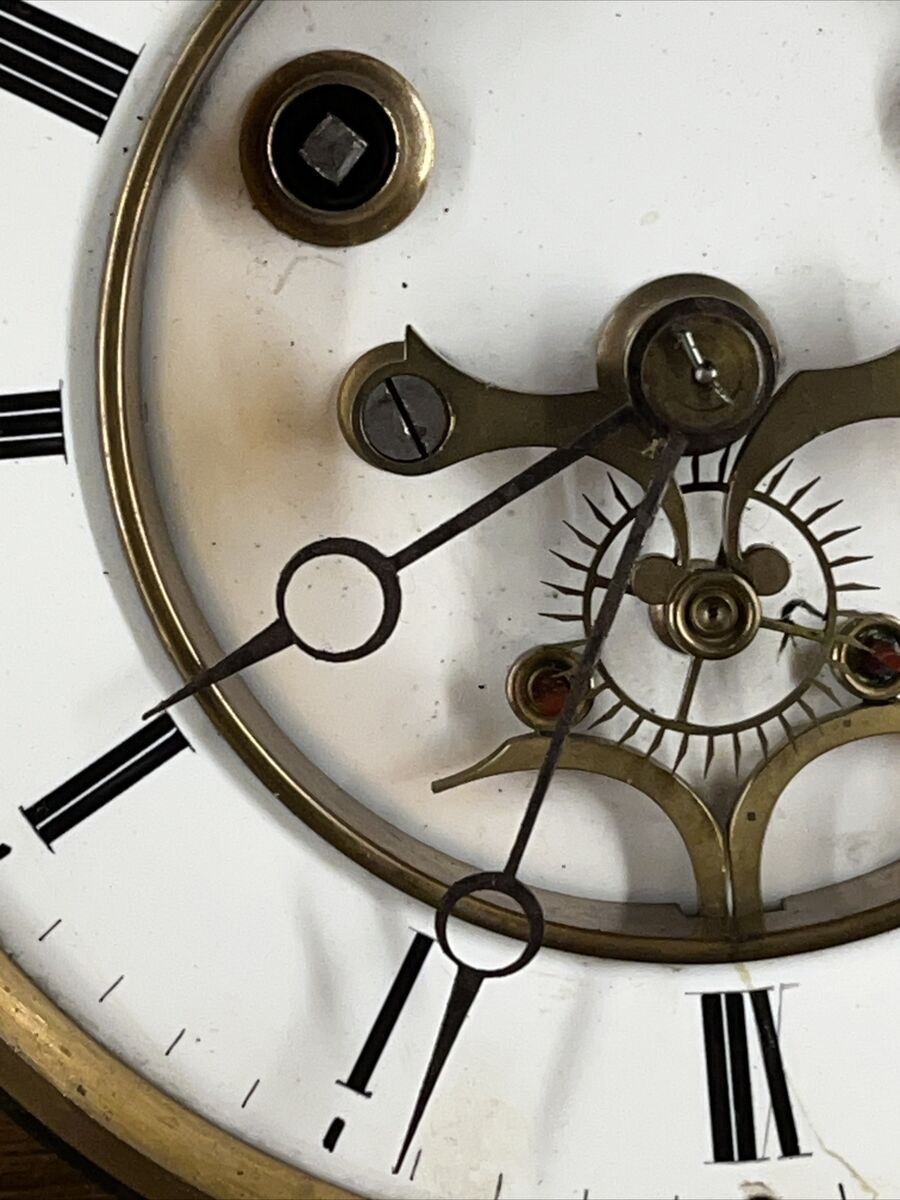This image presents an extremely zoomed-in, detailed view of the central workings of a large, wall-mounted clock. The clock face is dominated by a white dial featuring black Roman numerals for the hours, with significant markers every five minutes and smaller slashes indicating individual minutes. At the core, intricate brass machinery, gears, and complications are visibly integrated into the dial. The clock is adorned with two long brass hands—a minute hand and an hour hand—each characterized by a circular base from which a pointed arrow extends. The outer edge of the clock is encased in a light ash-colored wooden frame, adding to its classic, elegant appearance. Currently, the time indicated on the clock is 2:04.